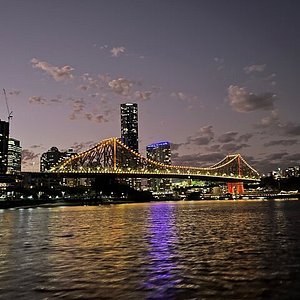This photograph showcases a picturesque twilight cityscape featuring a suspension bridge that stretches impressively over a body of water. The photograph is likely taken in San Francisco, capturing the iconic bridge adorned with lights that illuminate both above the top frame and along the roadway. A cityscape emerges prominently in the background with several high-rise buildings, including a notable purple building that casts a reflective purple glow onto the water. The sky is a mesmerizing mix of purples, bluish-grays, and hints of muted oranges and pinks, adorned with scattered gray and white clouds. The water in the forefront poignantly mirrors the city lights, adding an enchanting effect to the entire scene. The overall atmosphere is reminiscent of dusk, with the dim lighting providing a serene yet vibrant backdrop to this urban landscape.